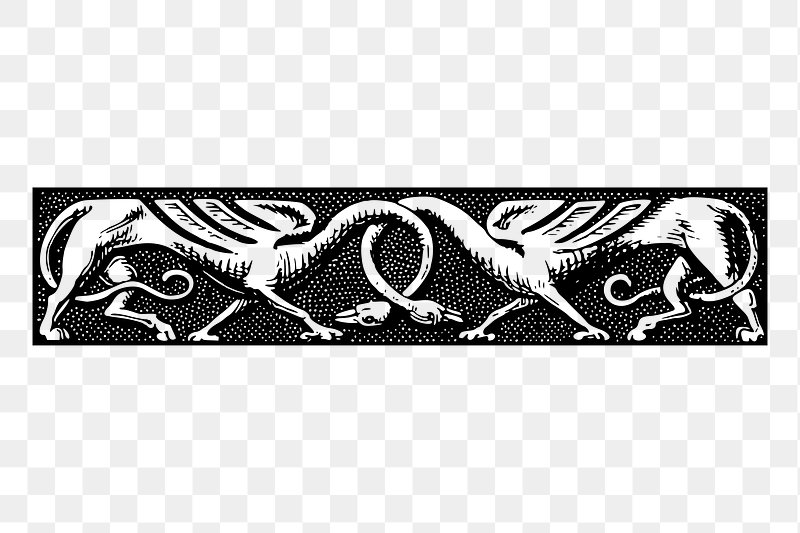This detailed illustration features two mythical creatures, rendered in black and white, set against a background of gray and white checkered pattern intended to represent transparency. The creatures, depicted within a long horizontal black rectangle with white dots, boast a fantastical hybrid design. 

Each creature displays the robust hindquarters of a lion, complete with muscular back legs and long, curving tails that weave through their legs. Their midsection is adorned with three wings, resembling those of a bird or dragon, fanning out in layered segments. Their elongated necks, reminiscent of a goose or dragon's, entwine intricately to form an oval shape, their heads facing downward and inward, creating a symmetrical, interlocked stance. The heads themselves are goose-like, featuring beaks and a predatory gaze. This hand-drawn image combines elements of mythical and real creatures, presenting a harmonious yet complex design perfect for a fantasy-themed banner or crest.